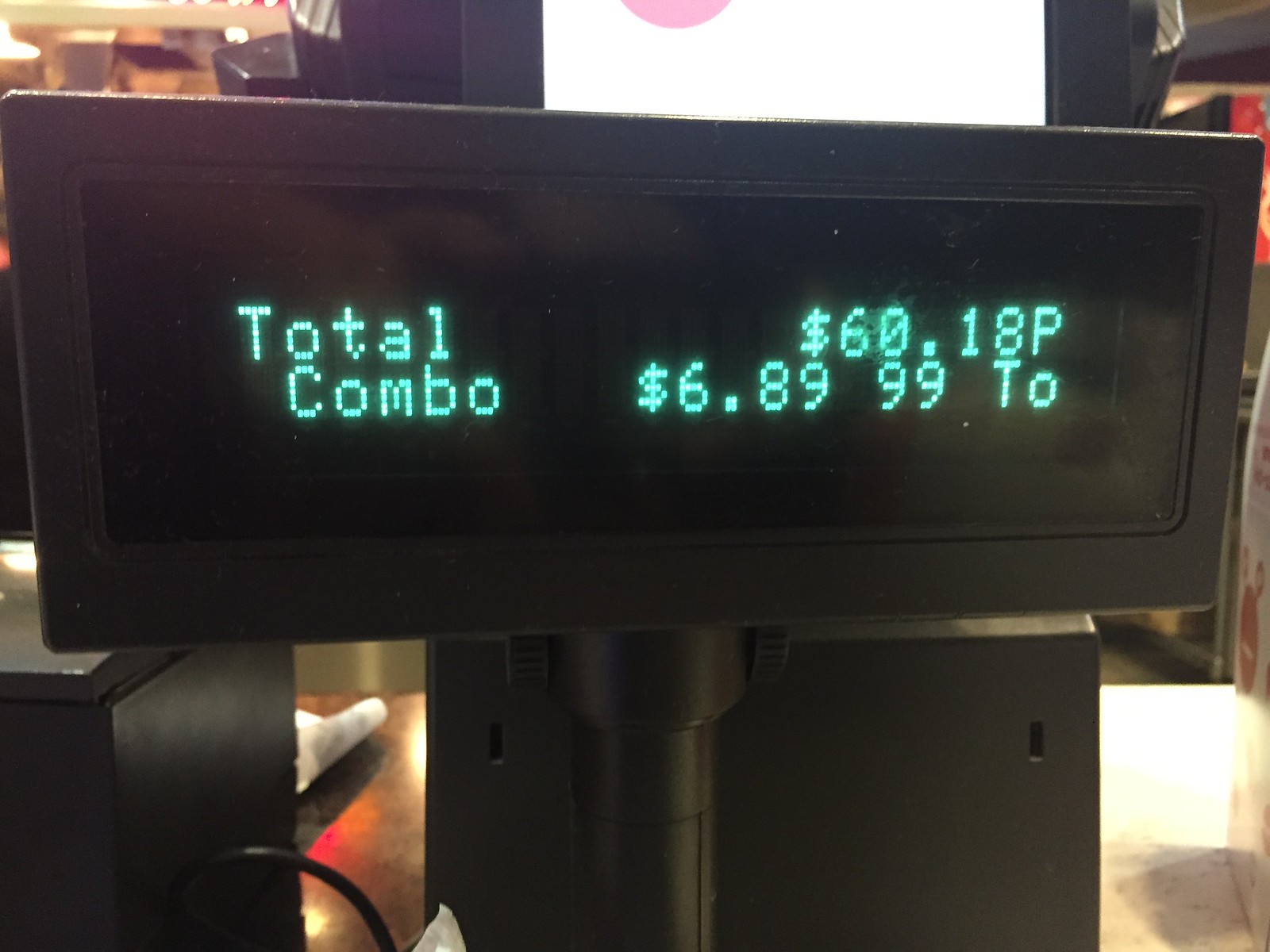The image depicts a checkout station featuring a rectangular digital readout screen atop a black cylindrical pole. The screen, oriented horizontally, displays neon green text and figures. On the right side of the screen, the word "Total" is visible, followed by "$60.18P." Beneath it, the word "Combo" is displayed with "$6.8999TO." To the left of the display, a black box with a cable protruding from it can be seen, alongside various indistinguishable background elements. Additionally, a white sign with a partial red circle is situated on the top left corner of the image, and some countertop space is present in the lower section.